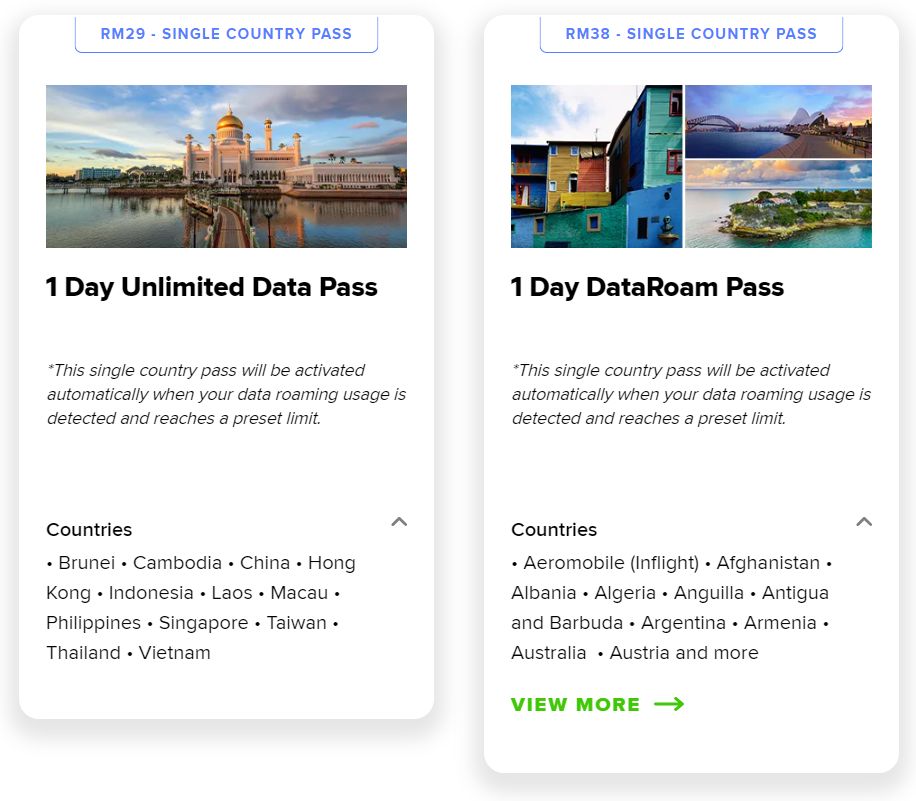This rectangular image, oriented vertically, features two side-by-side screenshots, each framed with a shadowed gray border. Both screenshots present travel-related passes.

The first screenshot features a white background with a blue-lined box at the top. Inside the box, in blue text, it reads "RM29 - Single Country Pass." Below the text is an image resembling the famous Taj Mahal, set against a picturesque scene with a lake in the foreground, a bridge, and various buildings surrounding it. Beneath the image, a bold statement reads "One Day Unlimited Data Pass." Further down, additional information explains that this single country pass will activate automatically when data usage reaches the preset limit. The list of applicable countries includes Brunei, Cambodia, China, Hong Kong, Indonesia, Laos, Macau, Philippines, Singapore, Taiwan, Thailand, and Vietnam.

The second screenshot closely mirrors the first in design, with a similarly shadowed gray border. At the top, against a blue-lined box, blue text announces "RM38 - Single Country Pass." Below, three smaller images feature vibrant buildings on the left and water landscapes on the right, suggesting more travel destinations.

This image likely serves as a comparative advertisement for two different travel data passes, providing key details and visual representations to potential users.